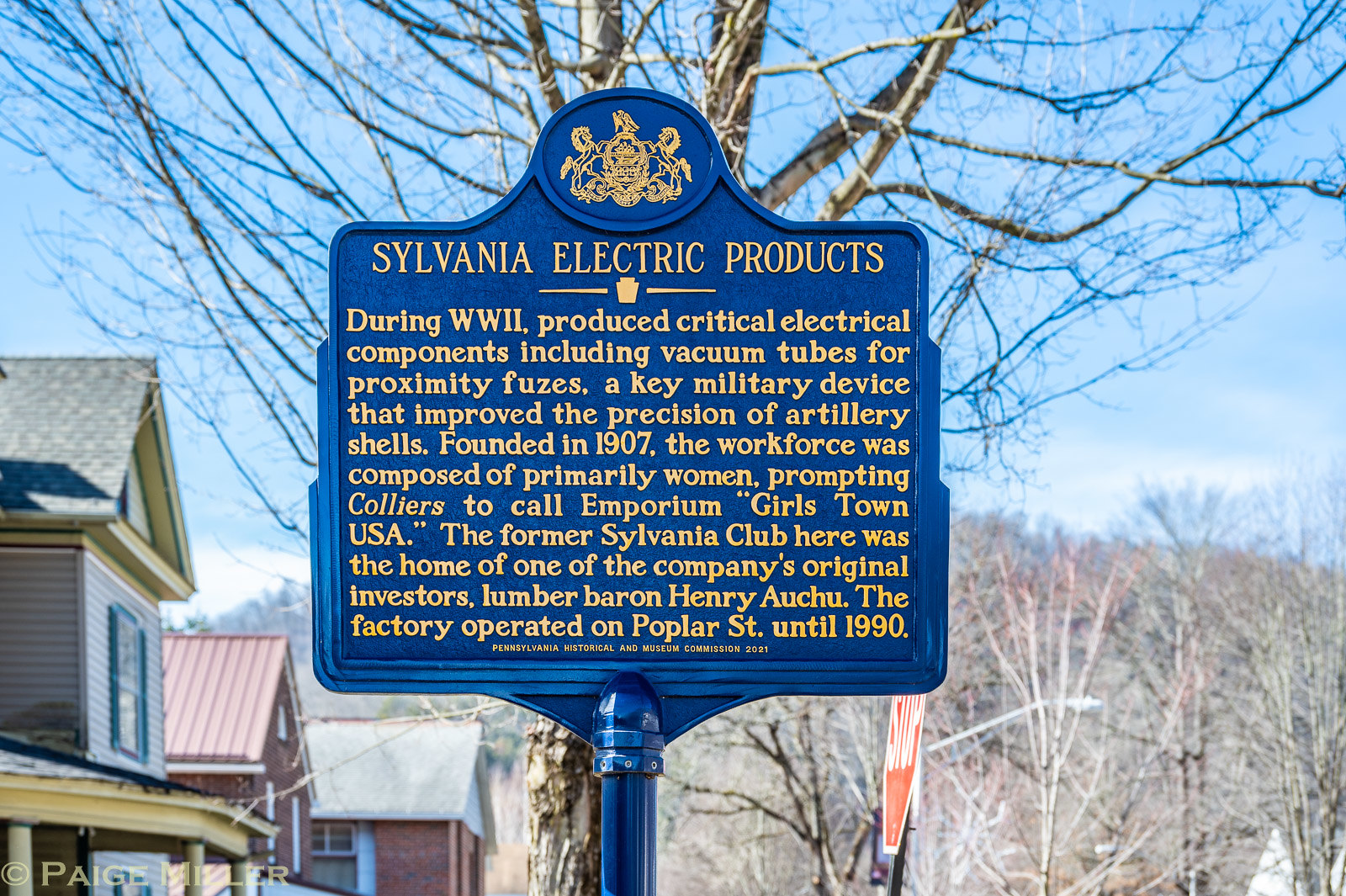The photograph depicts a blue, decorative metal sign with gold text mounted on a post. At the top of the sign is a circle featuring a gold coat of arms. Beneath that, in large letters, the sign reads "Sylvania Electric Products." The main text elaborates that during World War II, this company produced critical electrical components, including vacuum tubes for proximity fuses, which significantly improved the precision of artillery shells. Sylvania Electric Products, founded in 1907, utilized a workforce primarily composed of women, earning the moniker "Emporium Girlstown, USA." It mentions that the former Sylvania Club, situated nearby, was once the home of one of the company's original investors, lumber baron Henry L. Auchu. The factory operated on Poplar Street until 1990.

In the background, there is a bare tree, suggesting that the photograph was taken during the winter. Also visible are a series of trees and a hill in the distance. To the left of the sign is a stop sign, and behind it is a row of two-story wooden and brick houses typical of a small town's commercial area. The sky is blue and bright, illuminating the scene.